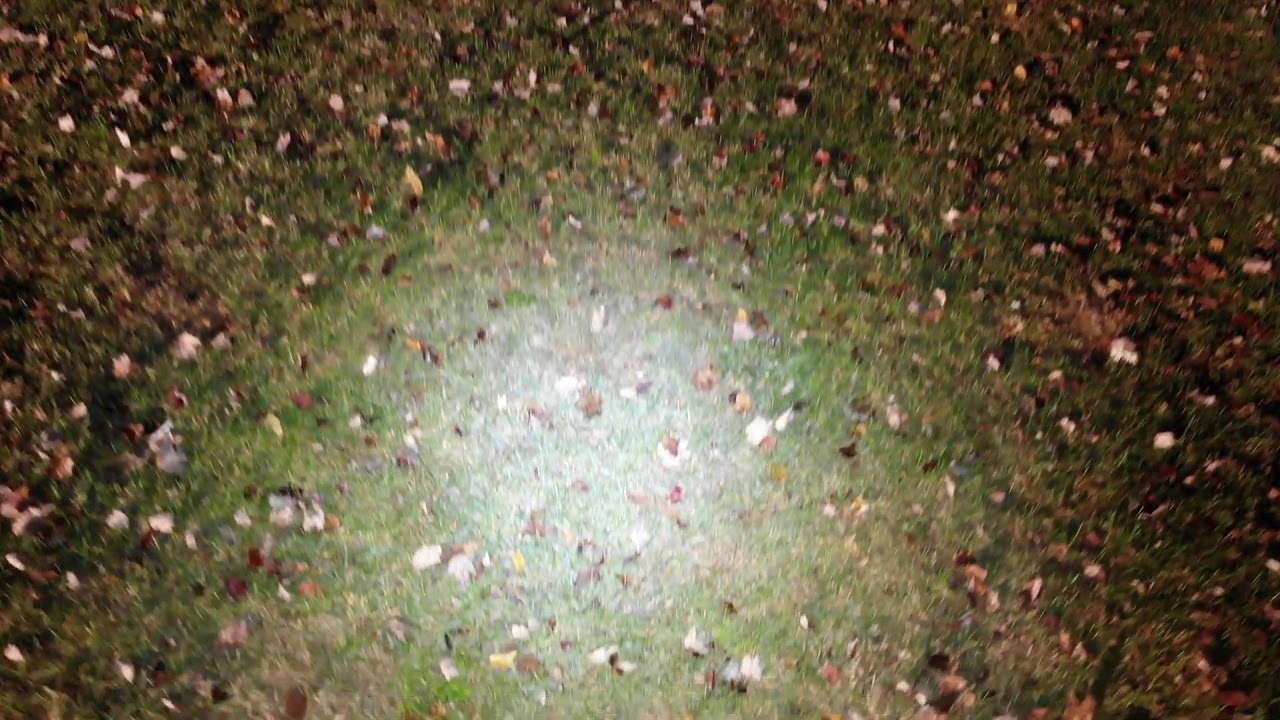A captivating image captures the ground illuminated by a bright, cold white light at the center, creating a stark contrast with the surrounding darkness. The photograph, taken from a standing position looking directly down, showcases a patch of green grass within this central illuminated area, with fewer leaves scattered across it. Beyond the reach of the light, the grass blends into a dimly lit, almost black background, with a thicker scattering of leaves in various shades of brown, yellow, and orange. The leaves appear concentrated and close to each other in the periphery, adding texture and color to the darkened surroundings as if highlighting the transition from light to shadow in this serene night or dimly lit setting.